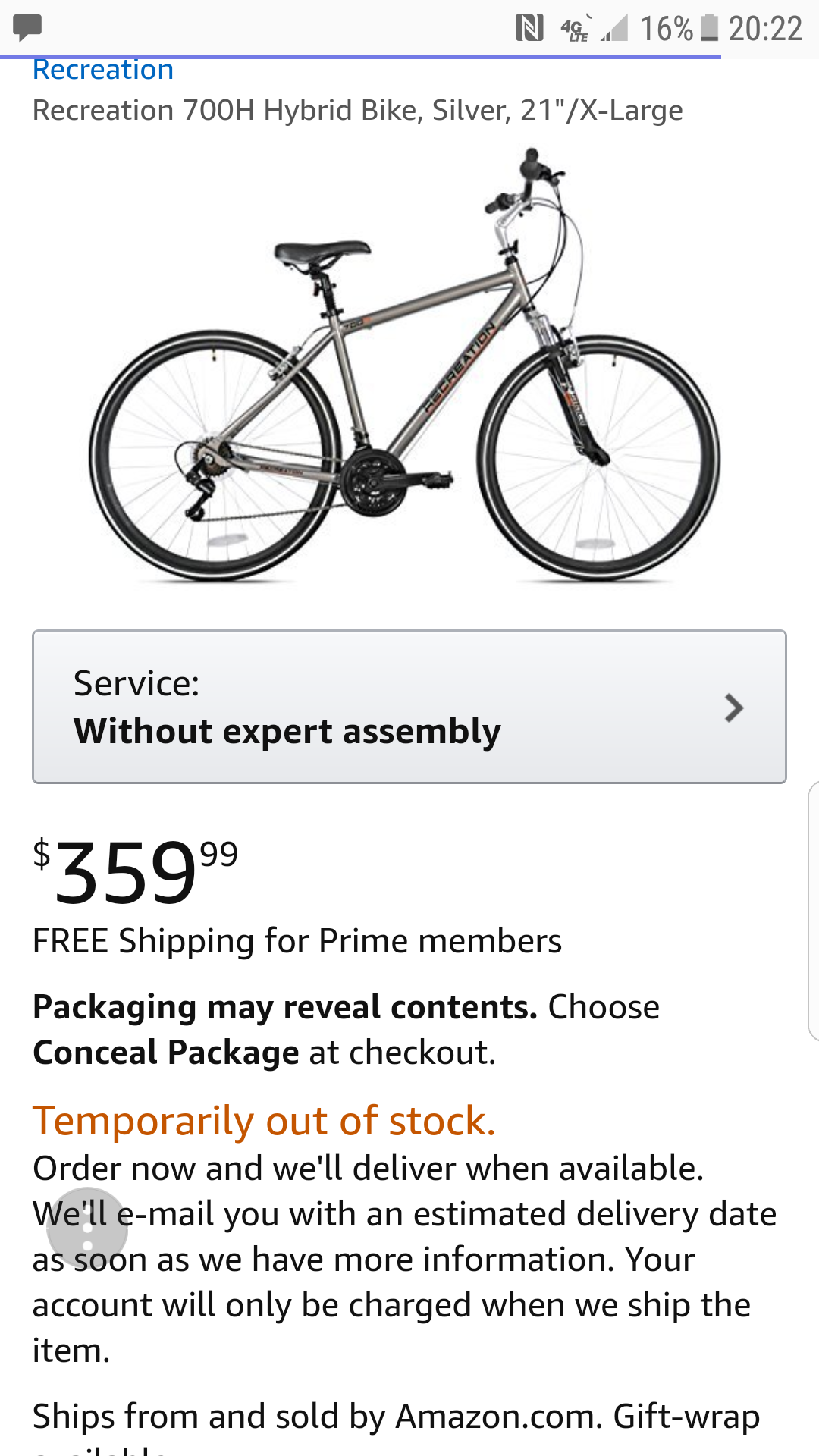A screen capture of a cell phone displays multiple details. The time on the phone reads 20:22 (8:22 PM) and the battery is at 16%. The device has a weak signal with only one bar of reception. The screen prominently features a listing for a "Recreation 700H Hybrid Bike" in silver, with a 21-inch extra-large frame. Accompanying the text is a clear image of the bicycle. The price is marked at $359.99 with free shipping available for Prime members. The listing includes a note that packaging may reveal the contents, and offers an option to choose a concealed package at checkout if the purchase is a gift. The bike is noted as "temporarily out of stock" in red text, with a message stating, "Order now and we'll deliver when available. We'll email you with an estimated delivery date as soon as we have more information. Your account will only be charged when we ship the item." The item is to be shipped from and sold by amazon.com, with an option for gift wrap visible but cut off.